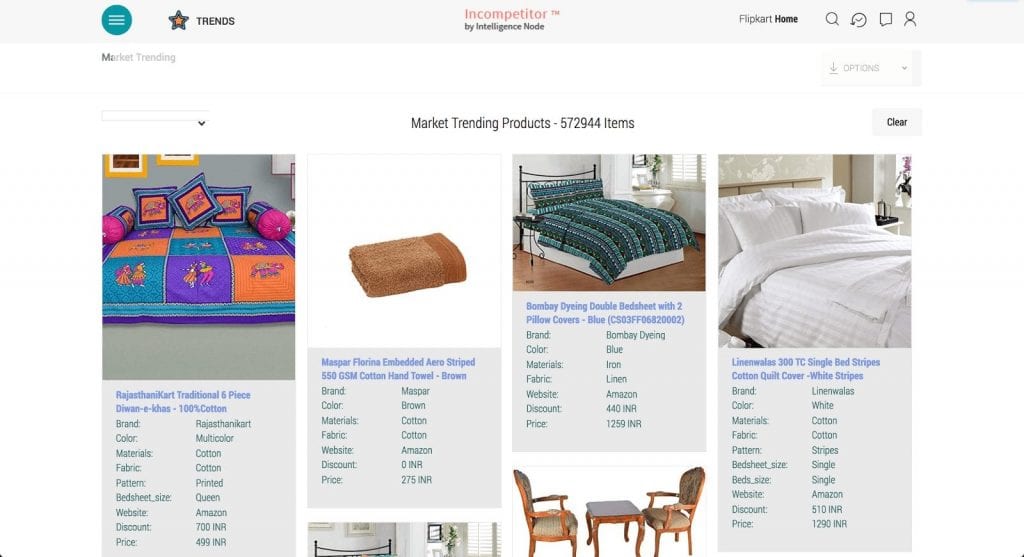Screenshot of the "Incompetitor" platform by Intelligence Node, displaying trending products on Flipkart, Amazon, and other e-commerce websites. The page is geared towards dropshippers, showcasing popular items and market trends to help sellers identify profitable products. The current count of market-trending items is a staggering 572,944. Featured products include a traditional six-piece, 100% cotton bed cover set with comforters and pillow covers, striped cotton hand towels in brown by Bombay Dyeing, a double bed sheet with two blue pillow covers, and a single bed striped cotton quilt cover reminiscent of hotel bedspreads. Also displayed are table chairs and another bed set. This comprehensive platform aggregates data from various sources, making it a valuable tool for online sellers looking to stay ahead of the competition.